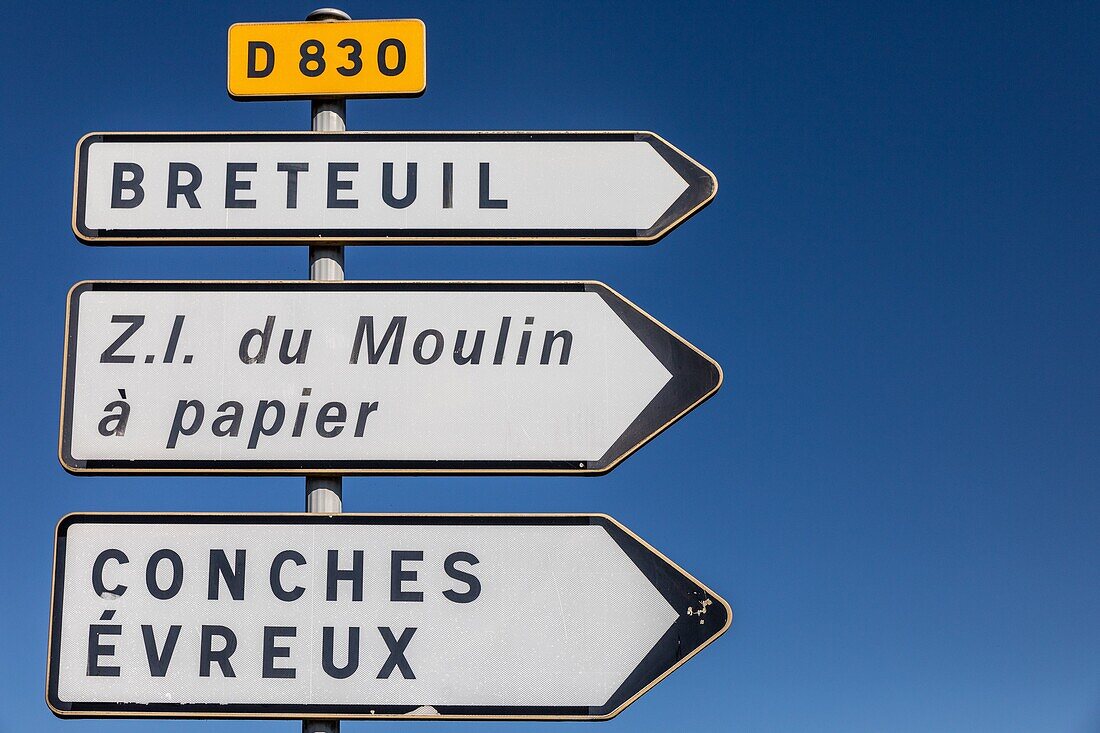The photograph captures a signpost set against a deep navy blue sky. The signpost holds four distinct signs arranged vertically. At the top of the pole is a dark yellow square sign with black text that reads "D830." Below this, there are three white signs, each with black text, pointing to the right. The first sign is long and rectangular, with the word "BRETUIL" (spelled B-R-E-T-U-I-L). The second sign, slightly larger and ending in an arrow shape, reads "ZI DU MOULIN A PAPIER." The third sign is similar in size to the second and contains the words "CONCHES" and "EVREUX" (E-V-R-E-U-X). All signs direct towards the right side of the image, providing clear navigational information.